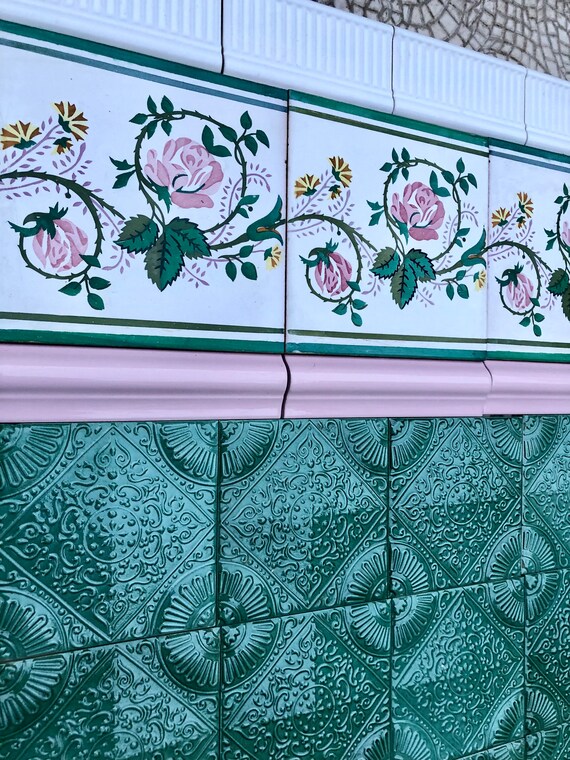The image shows a vertically aligned, close-up view of a decorative interior wall tiled in an intricate, multi-patterned design. The top section features white rectangular tiles, each with vertical grooves, giving a textured appearance. Just below these are square, white ceramic tiles adorned with floral designs, including pink roses, green vines, and leaves, with the added detail of a yellow flower on the left. These tiles are bordered at the top and bottom by dark green lines. Following these are rectangular tiles in a soft pink hue, acting as a border strip. Below the pink tiles are shiny green tiles with intricate, old-fashioned patterns, including diamond designs and circular motifs at the corners. The overall arrangement showcases a detailed and elegant floral theme, indicative of sophisticated interior decoration.